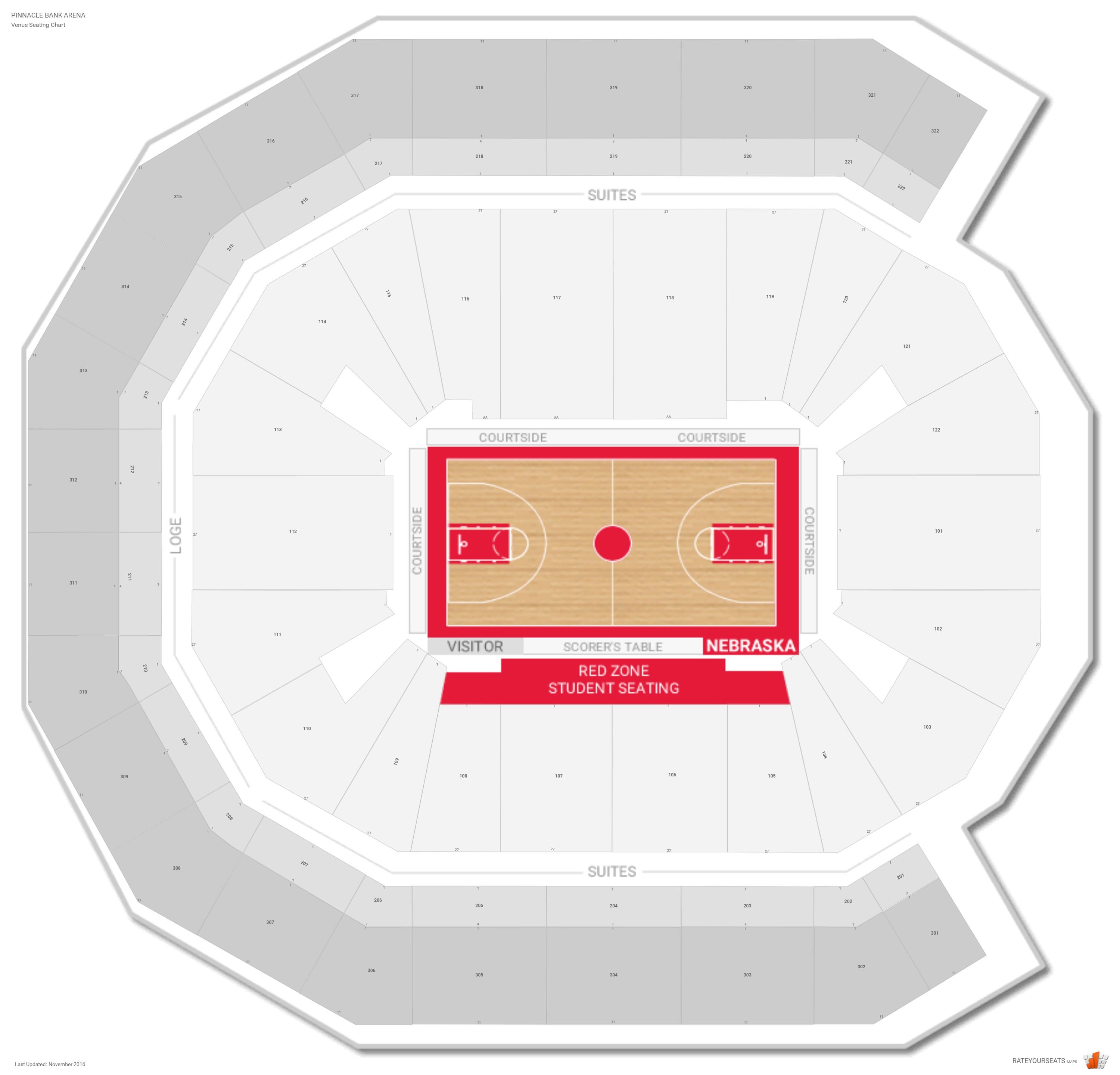**Detailed Captivating Caption:**

This image showcases a comprehensive seating map for the Pinnacle Bank Arena, highlighting its layout for a basketball event. The background is a clean white, making the detailed, gray-outlined sections and text easy to distinguish. In the upper left-hand corner, small gray text reads "Pinnacle Bank Arena Venue Seating Chart."

At the heart of the diagram, a meticulously detailed basketball court is depicted with visible wood panel flooring, alongside essential markings like the half-court line and other standard basketball lines painted in white. The court is bordered by a striking red outline.

At the bottom of the court, there’s a designated "Red Zone Student Seating" area. The word "Nebraska" is prominently displayed in bold red text on the bottom right side of the court, opposite from the visitor's section. Central to the court is the scorer's table. Surrounding the court on the other three sides, the map labels "court side" seating, indicating premier viewing spots.

The arena seating is organized into various levels: the lower level closest to the court, followed by the loge and suite level, and the subsequent second and third tiers of seating. These levels provide a structured hierarchy for the venue, ensuring a range of viewing experiences for attendees.